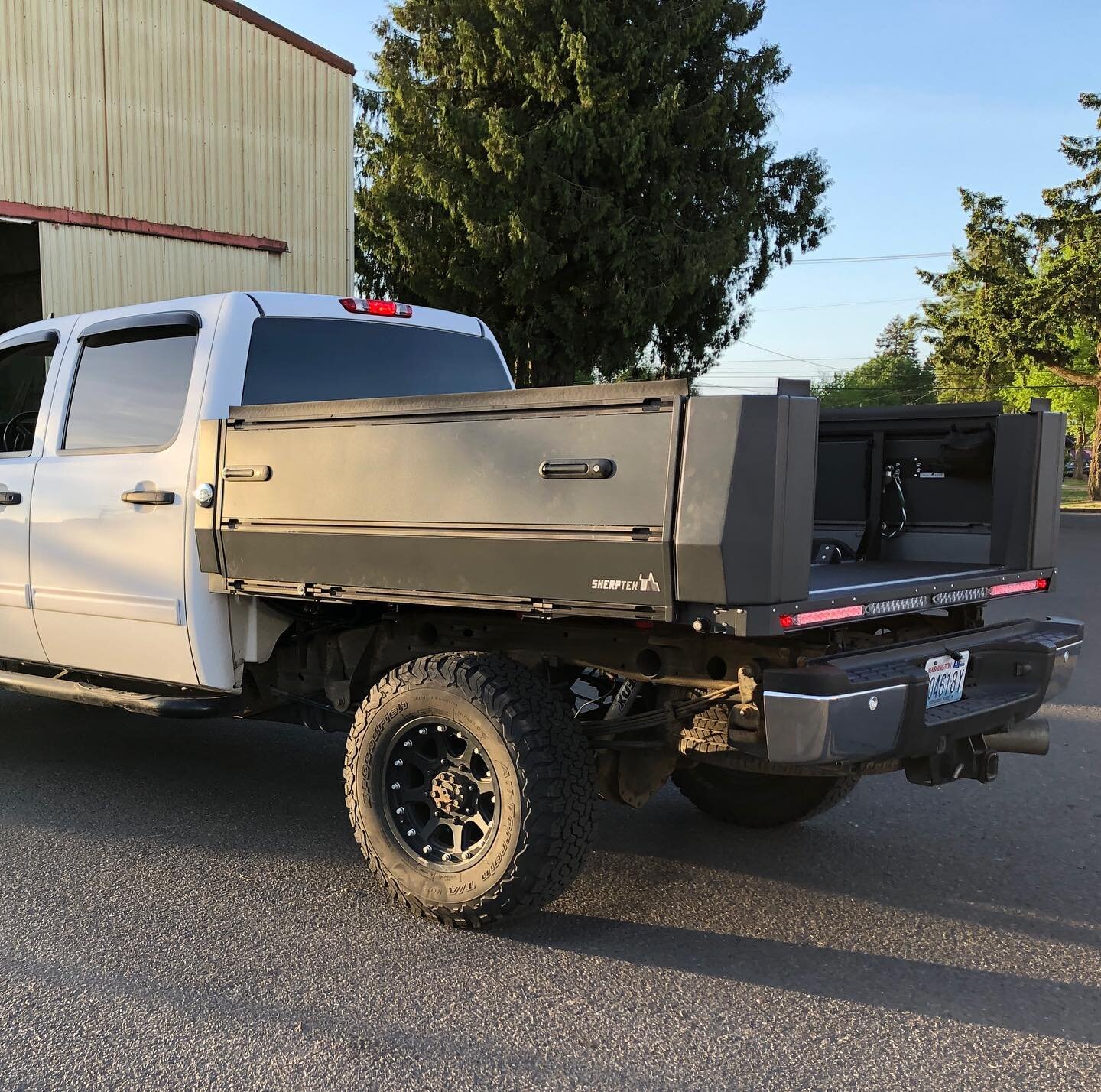This square photograph captures a white, four-door pickup truck parked in front of a tan tin building with red accents that resembles a garage or shed. The truck, which appears to be a modified Chevy, has had its original bed replaced with a custom black flatbed utility feature, giving it a work truck appearance. The vehicle has a lift kit or appears elevated due to the custom back, and it bears a Washington State license plate, indicating its local origin. The front portion of the truck is cut off on the left-hand side, showing only the back half and a three-quarter view of the driver's side and passenger side doors. The truck is parked on an asphalt surface, with bungee cords visible in the bed. The scene is set on a sunny day with a clear blue sky, and the background features multiple trees and power lines. The building looks slightly worn, as if it could benefit from a power wash, but it is not old.